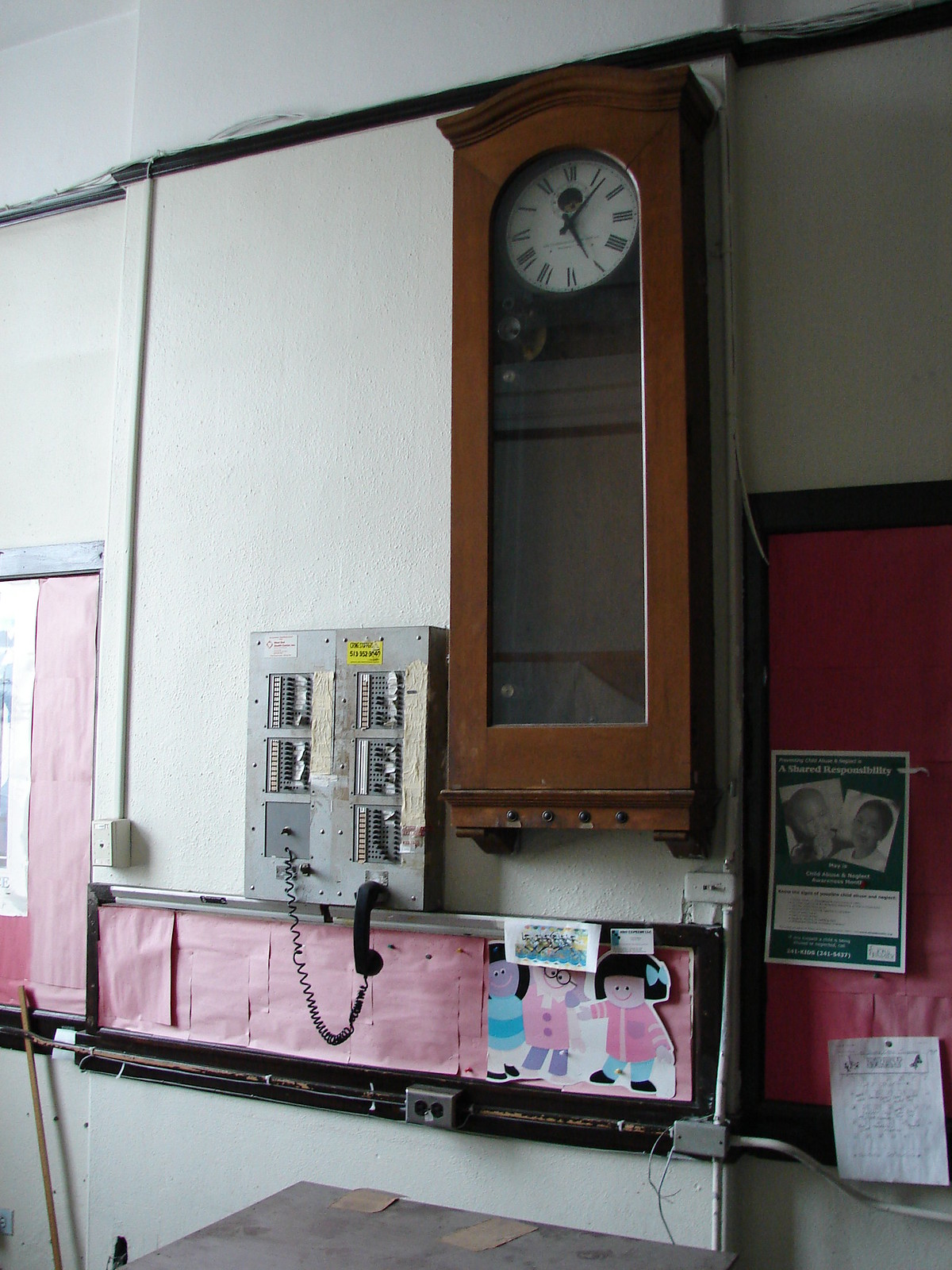This detailed color photograph captures a school classroom scene dominated by a white-walled backdrop. Central to the image is a small old-style analog clock encased in dark wood, with a white face displaying black Roman numerals and black hands, enclosed behind a curved glass door. The time shown is approximately 5:07. Adjacent to the clock is a circuit board and an attached black telephone with a curly black cord, suggesting a possible PA system setup. The board has a silver finish with a dangling black foam component. Below this assembly is a gray, large electrical socket. The wall also showcases a bulletin board framed in black and lined with red construction paper, adorned with children's drawings of girls in red coats, indicating a vibrant and creative classroom atmosphere. A dusty dark wood desk adds a touch of antiquity to the scene.